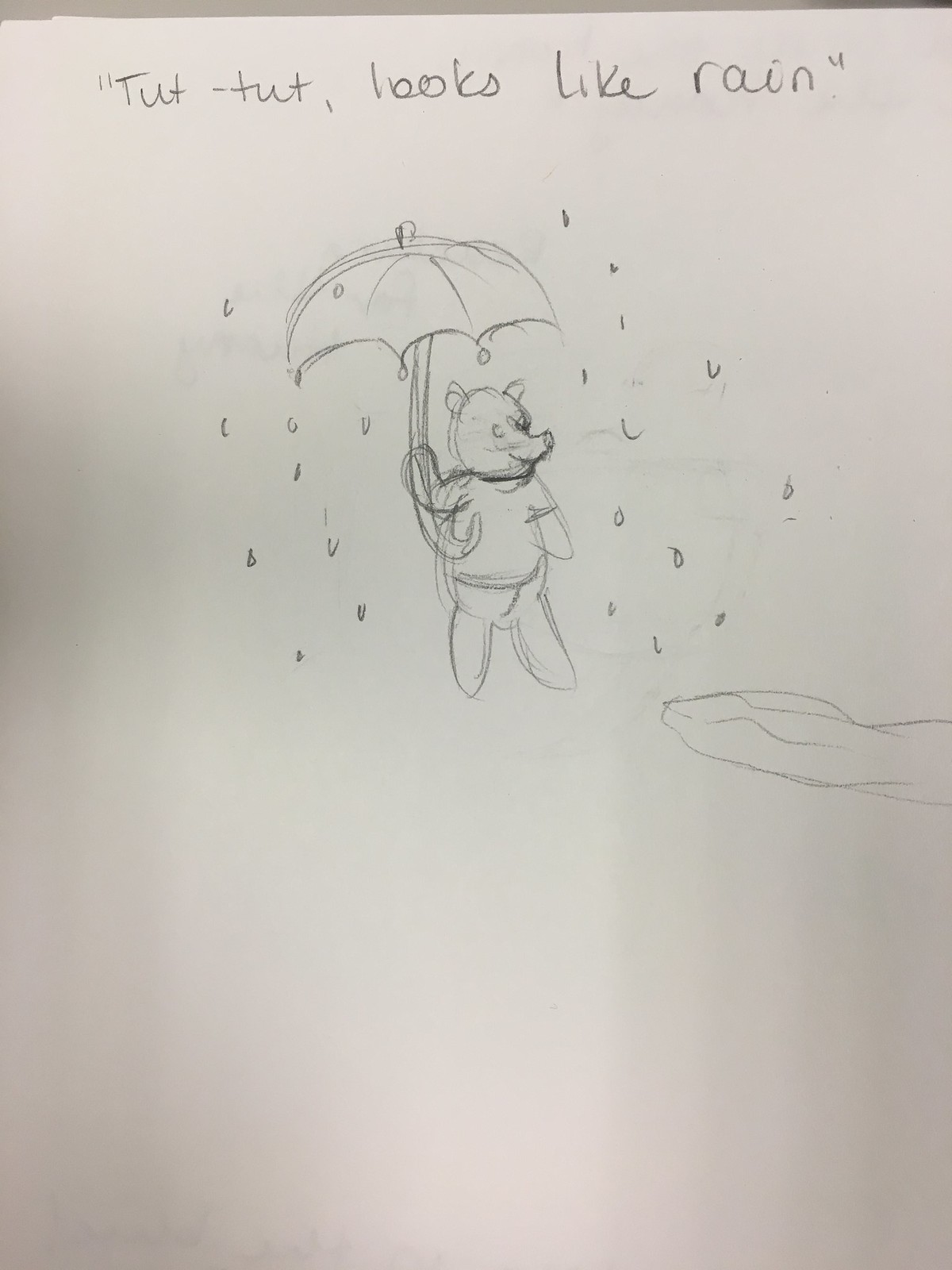This detailed, monochrome pencil sketch is on a piece of off-white paper, with a few shadowy areas in the left or right corners. The image features a character resembling Winnie the Pooh, standing upright and facing to the right. He is depicted with a slightly exaggerated snout and wears a t-shirt, but no pants, consistent with his usual appearance. Winnie the Pooh holds an umbrella in his right paw, which is open and detailed with traditional umbrella lines and a knob at its center. Surrounding him are rain droplets, with some resembling traditional teardrop shapes and others drawn as upside-down U's, creating a sense of varied rainfall. Below and to the right of Pooh is an elongated, squiggly line suggestive of a puddle. Above the character, in handwritten pencil text, is the quotation: "Tut, tut, looks like rain," with distinctive, slightly cursive O's in the word "looks" that almost resemble glasses. The sketch occupies the upper half of the page, while the lower half remains blank, save for the subtle shadowing.